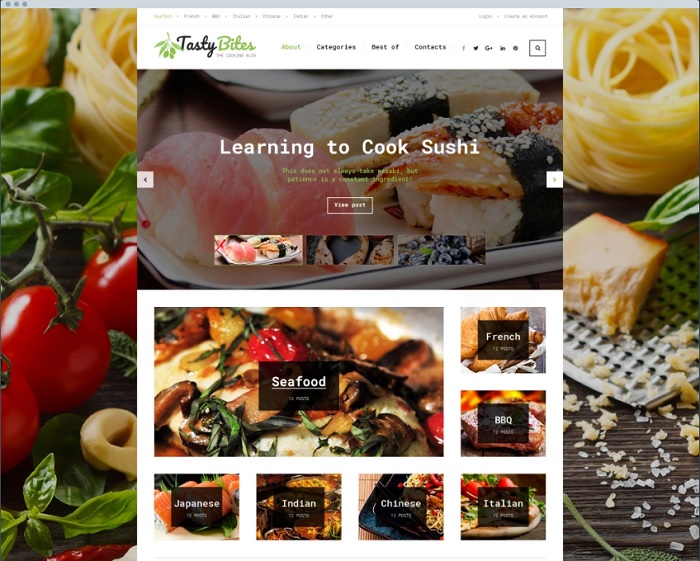The image is a horizontally rectangular photo featuring a vibrant background of different culinary delights. In the upper right corner, a delectable plate of pasta is displayed, and directly below it, a block of fresh cheese rests atop a cheese grater. To the left of the cheese, a cluster of vine-ripened tomatoes adds a pop of color.

Taking center stage is a vertical rectangular section superimposed over the food background, showcasing a tantalizing array of dishes. In the upper left corner of this section, the words "TastyBites" are prominently displayed on a white background, with "Tasty" in a dark font and "Bites" in a light green font. Preceding "TastyBites" is a logo depicting a green stem with leaves and some circular elements.

At the top of the vertical section, a navigation bar features categories in different fonts. "About" is highlighted in green, followed by "Best Of" and "Contacts" in a darker font. Below this, a faint image of sushi serves as the background for bold white text that reads "Learning to Cook Sushi." Beneath this title, there is green text that is difficult to read, stating something like "This does not always take."

Further down, a thick white horizontal area creates distinct sections in the central part of the image. This area features bolded white lines separating various sections. The first horizontal section is labeled "Seafood" in underlined white font. To the right, a vertical column showcases categories such as "French," "BBQ," and "Italian," each accompanied by food images such as croissants under "French." 

At the bottom of the vertical section, additional categories are listed in a black horizontal rectangle with white text, including "Japanese," "Indian," "Chinese," and a reiterated "Italian." Each category is paired with corresponding food images, enhancing the rich, global culinary showcase.